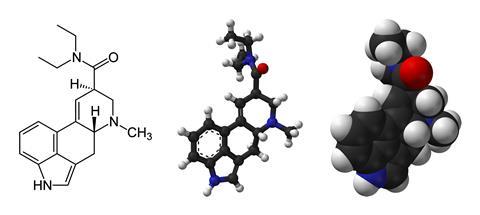The image showcases a detailed 3D rendering of a chemical molecular compound, presented in a three-part collage against a white background. On the left, we see the traditional chemical composition diagram, consisting of lines and letters such as N, O, H, C, depicting the bonds in a standard notation. The central image presents a two-dimensional molecular model, featuring small white, blue, and red circles connected by thin black lines, forming a network of black circular rings with white protrusions, and a notably prominent red sphere. To the far right, we observe a vivid three-dimensional representation, where differently colored spheres (black, white, red, and blue) are interconnected, creating a tangible, spatial model that vividly illustrates the compound's structure within a black framework. This triptych captures the same chemical compound in its various forms, from theoretical diagrams to intricate 3D models, demonstrating the transition from abstract representation to physical visualization.